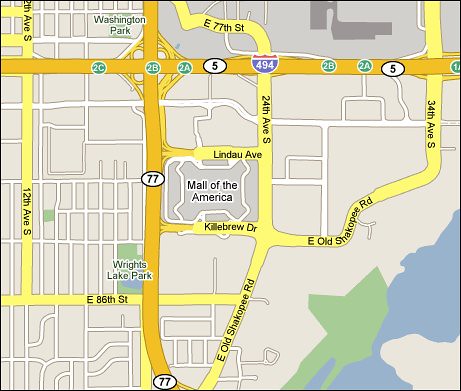Screenshot of a detailed street map designed for navigation, highlighting roads and major intersections. At the center of the map is a large area labeled "Mall of America." To the right of the Mall of America is a network of roads, prominently marked in yellow. The vertical road immediately to the right of the mall is identified as 24th Avenue South. Above this, running horizontally, is a significant highway labeled as both Interstate 494 and Highway 5.